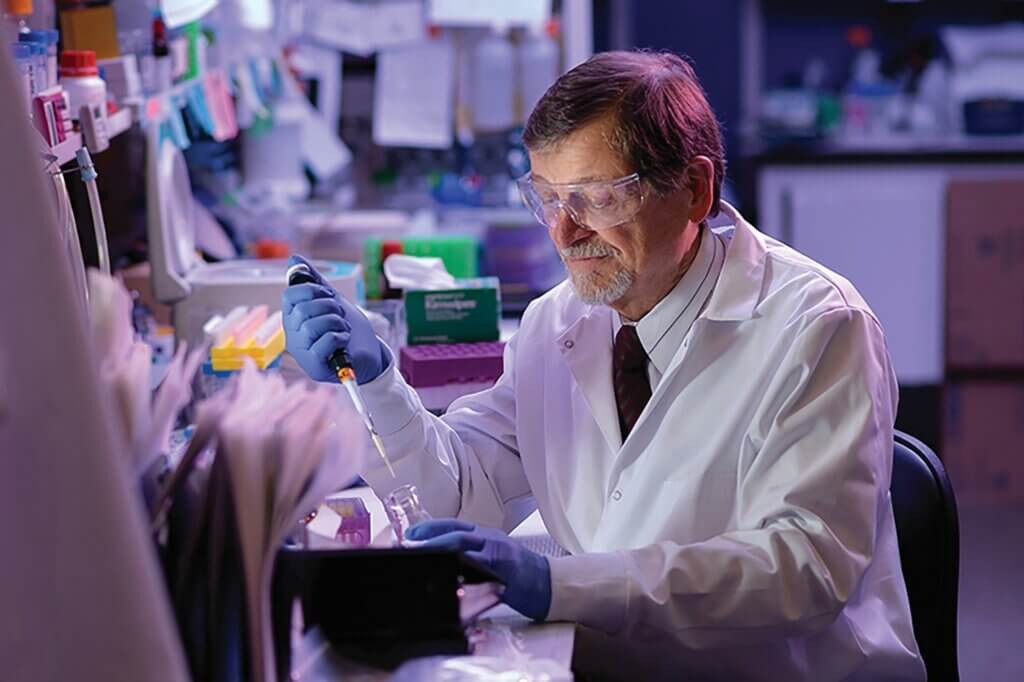This detailed photograph captures an older male scientist or laboratory worker engrossed in his work inside a bustling lab space. He has short dark brown hair complemented by a gray beard and mustache. His eyes are protected with clear plastic safety glasses, and he dons a white lab coat over a long-sleeve white shirt that features a distinctive black stripe around the collar. A black tie completes his professional attire. He is seated in a black chair at a cluttered desk, wearing blue latex gloves. In his left hand, he holds a clear glass test tube, while his right hand maneuvers a dropper or suction device, possibly inserting liquid into the tube. The laboratory background is slightly blurred but reveals an array of scientific instruments, bottles, tubes, and essential lab supplies. A collection of paper files stands upright on the desk amidst various other laboratory items, including what appears to be a box of tissues, underscoring the busy and crowded nature of the workspace.